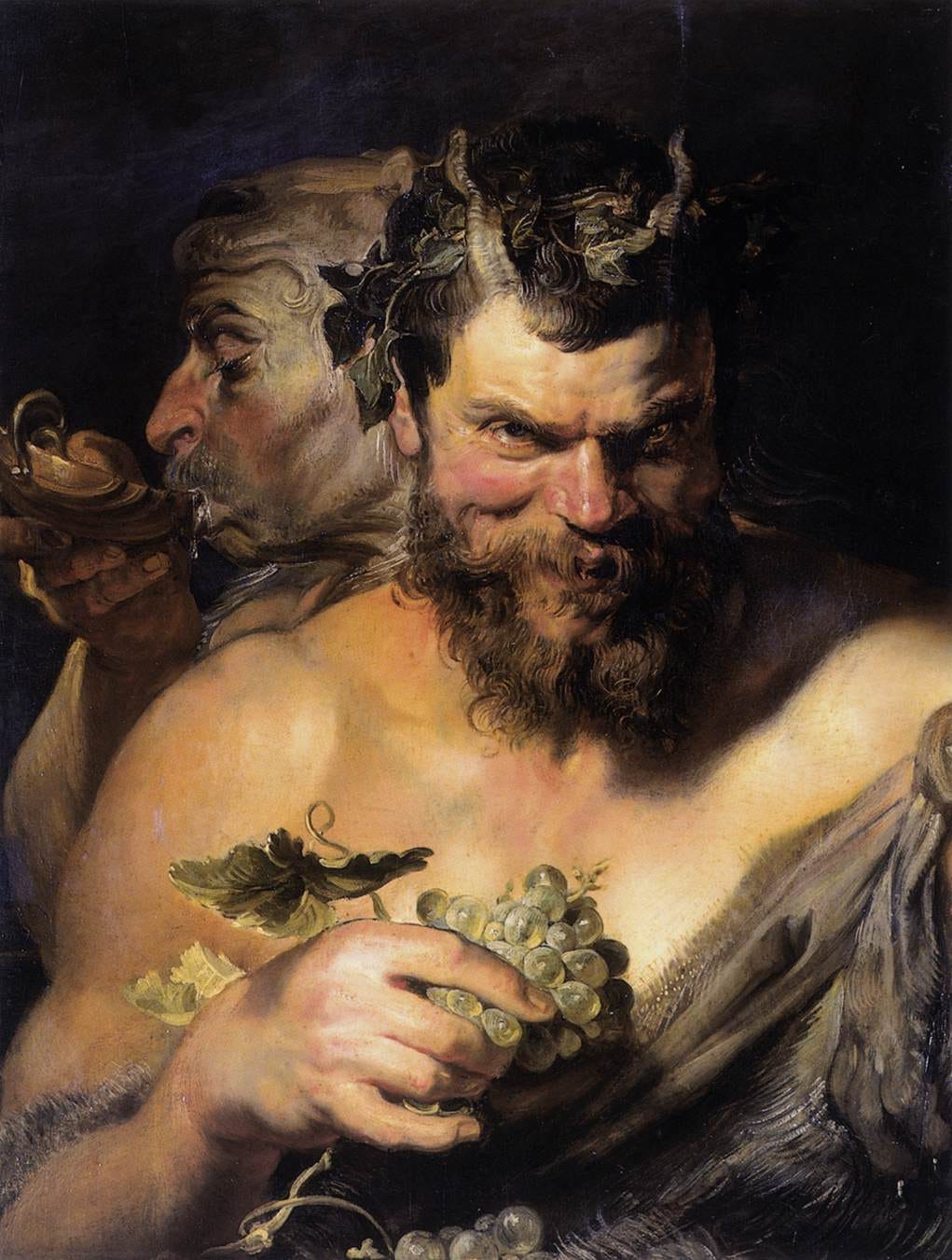This detailed painting, rendered in a realistic Renaissance style with a predominantly black background accentuated by a purplish-gray highlight at the top, features two male characters. The central figure, facing the viewer, is a large man with exposed upper chest and a fur-like toga draped over his right shoulder. He has brown curly hair, a curly beard, a mustache, and two small horns protruding from his forehead, angling backward. His cheeks and nose are visibly flushed red, and he wears a wreath of green leaves around his head. His white skin contrasts with his intense, menacing expression as he gazes up and to the right. In his right hand, he holds a bunch of green grapes with attached leaves and vines.

Behind him, partially shrouded in shadow, is a second man with a pale complexion and white hair. He has a white beard and a dark orange nose. This figure is turned to the right, focusing downwards as he sips from a small dish that resembles a brown shell, adorned with a little greenery. Both characters appear to be wearing garments made from fur. The painting’s intricate details and shadow play create an intense, captivating scene.